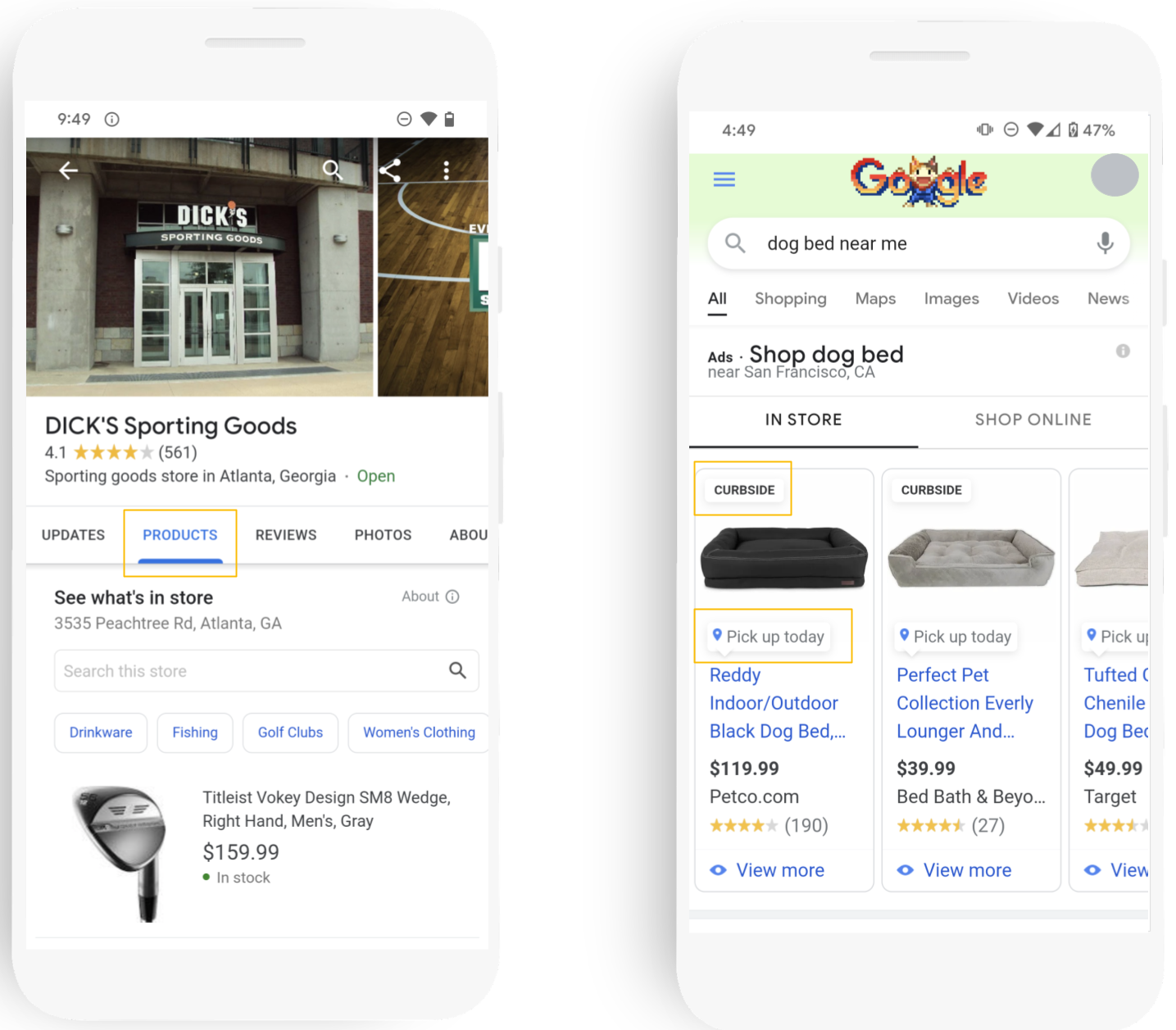In the first image on the left, an Android phone screen displays a search result for Dick's Sporting Goods located in Atlanta, Georgia. The store is currently open and has garnered a rating of 4.1 out of 5 stars from 561 reviews. The screenshot highlights a product listing for the Titleist Vokey Design SM8 Wedge, a men's right-hand gray golf club, which is priced at $159 and is currently in stock.

The second image on the right, also taken from an Android phone, shows a Google search results page for "dog bed near me." The search results are tailored to the San Francisco, California area. The top result is a ready indoor/outdoor black dog bed available at Petco for $119. The second result is a gray dog bed from Bed Bath & Beyond, priced at $40. The third result is a dog bed from Target.